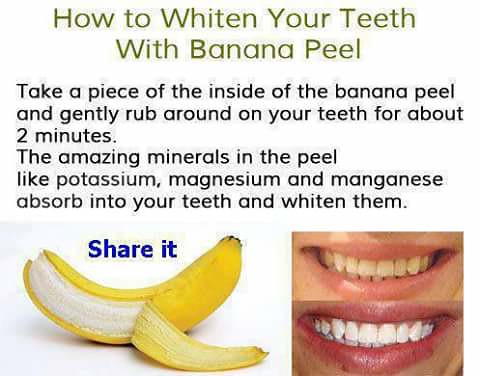The image features a white background with several elements centered and aligned for clarity. At the top, a heading in dark green text reads, "How to Whiten Your Teeth with Banana Peel." Below this heading, black text provides a description: "Take a piece of the inside of the banana peel and gently rub around on your teeth for about two minutes. The amazing minerals in the peel, like potassium, magnesium, and manganese, absorb into your teeth and whiten them." Beneath this explanatory text, there are three pictures: on the left, a partially peeled banana with the words "Share it" written in blue above it, and on the right, two before-and-after images of human teeth— the top showing yellowish teeth and the bottom displaying noticeably whiter teeth. This image appears to be an informational graphic, possibly for an advertisement or presentation, highlighting the natural teeth-whitening benefits of banana peels.